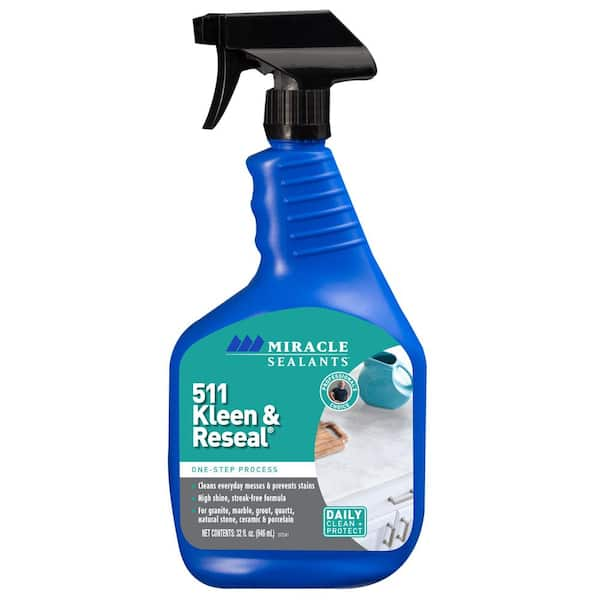This image features a spray bottle isolated against a transparent background. The spray bottle is designed with a sleek, ergonomic shape, beginning with a slim neck that broadens into a rounded square body. The bottle is primarily blue with a black top that includes a functional sprayer cap that screws securely into the bottle.

The label on the bottle is substantial, covering most of its rounded square body. The label is visually segmented into three horizontal sections: a green top portion, a white stripe in the middle, and a gray bottom section. 

At the top of the green section, the text reads "Miracle Sealants," followed by larger white letters spelling "5-1-1 Clean and Re-Seal," where "Clean" is distinctively spelled with a 'K' as "Klean." The white stripe underneath carries the text "One Step Process."

The gray section at the bottom contains a bulleted list of information marked by three green bullets lined vertically. The white text accompanying the bullets is not legible.

To the right side of the label, there is a visually engaging half-circle graphic depicting a pristine white countertop with matching white drawers in the background.

Additionally, situated in the bottom right corner, between the gray section and the half-circle graphic, is a square box containing the text "Daily Clean and Protect."

Above this square, there is a circular emblem with a green border and an obscured image in the center, the details of which are not clearly visible.